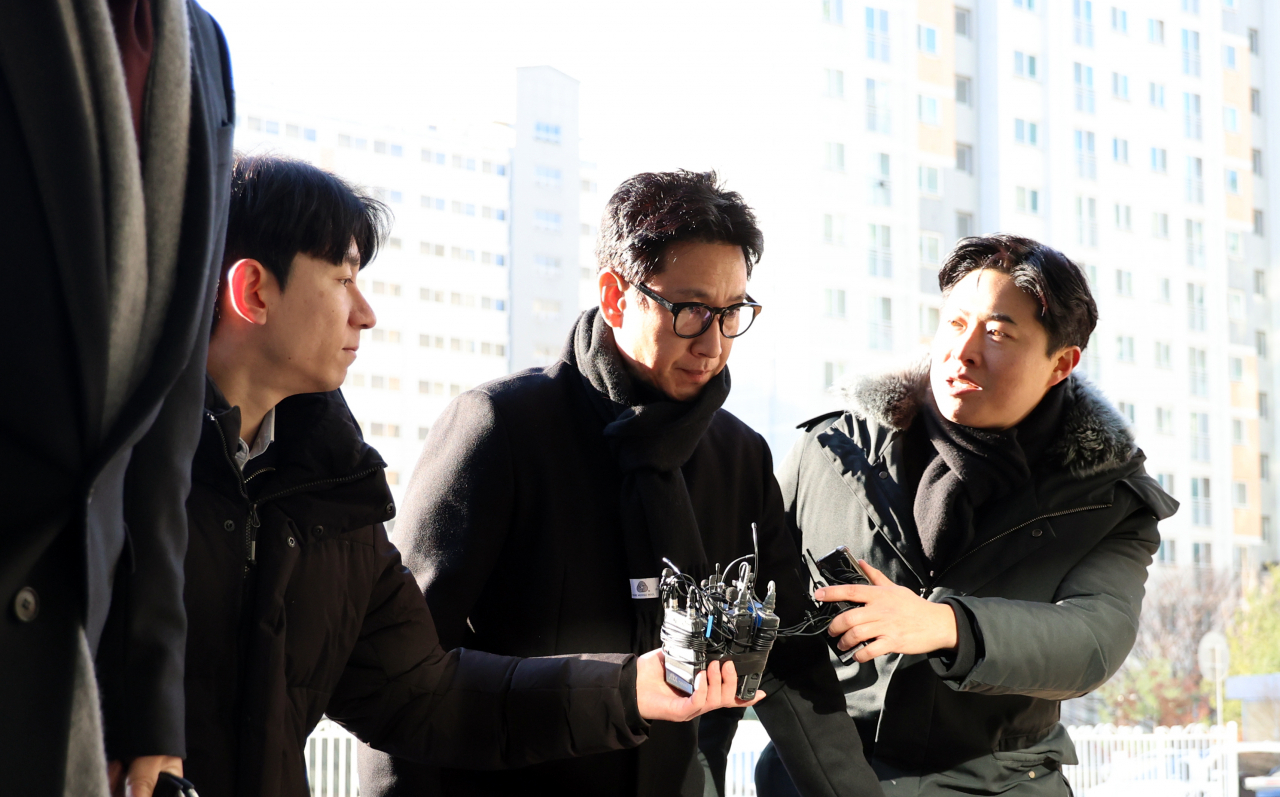The photograph showcases a close-up, horizontal shot of three Asian men, who appear to be standing outdoors in an urban setting during the daytime. All three men are dressed in cold-weather clothing, including dark jackets and scarves, suggesting a chilly environment. The man in the center is wearing dark-brimmed glasses and a black scarf, with short black hair. He seems to be disengaged, staring off to the right, while the other two men appear to be attempting to engage him in conversation. 

To the left, one man is holding a small mechanical device, possibly a deactivated bomb, with wires extending from it. This device could alternatively be interpreted as a tool or component. The third man, on the right, has a phone-like object in his hand, which may be a recorder or microphone. The backdrop of the image features high-rise buildings, each approximately ten floors in height, filling much of the background and emphasizing the urban locale. The colors in the image include black, gray, light green, white, beige, and tan, adding to the wintery and industrial feel of the scene.